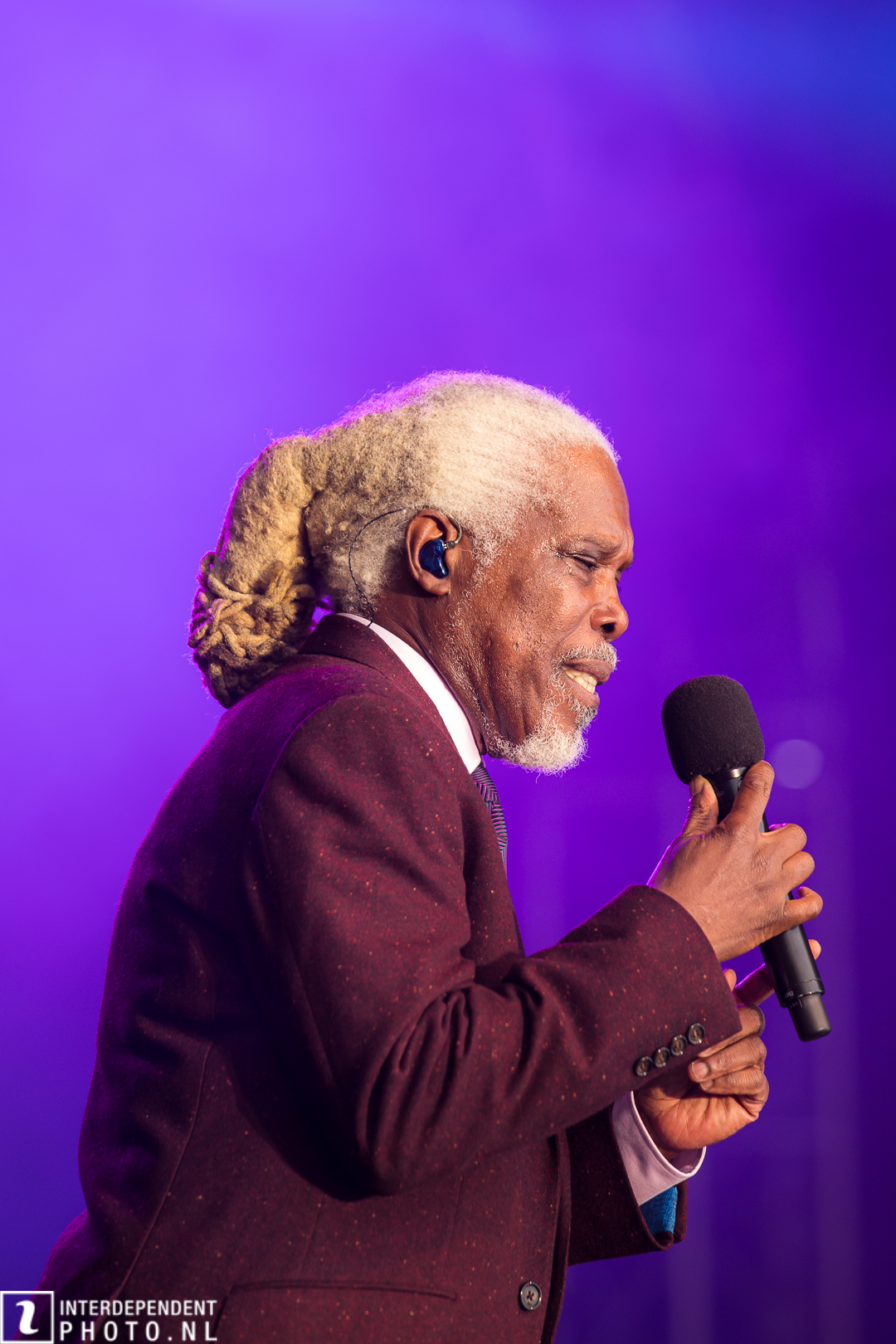The image shows a distressed-looking, older African American man on a stage with a purple backdrop. He has dark skin and white hair pulled back into a large, dreadlock-like ponytail. Wearing a burgundy or dark red suit jacket with four buttons on the wrist and additional buttons along the chest, he is also dressed in a white collared shirt and a tie. The man holds a large, fuzzy microphone with both hands and has a blue earpiece wire visible from his ear. His eyes are closed, suggesting he might be deeply engaged or performing, possibly delivering a speech or singing. In the bottom left of the image, "interdependentphoto.nl" is noted in white text.